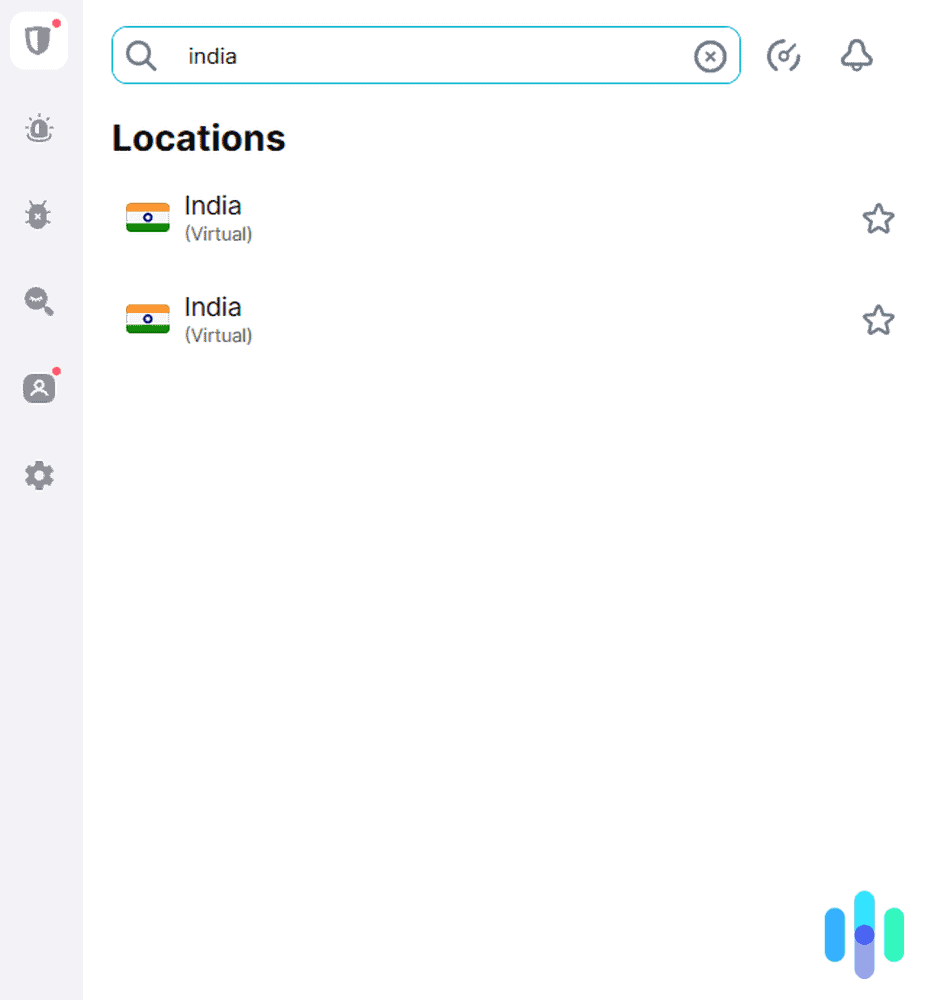The image is a screenshot displaying a user interface. On the left side, there is a vertical grey bar consisting of six elongated buttons. The first button, highlighted with a white box, is a grey shield icon featuring a small red dot near its top. Below this shield icon is a white siren icon, followed by a bug icon, a magnifying glass icon, a person icon with a red dot above it, and finally, a gear icon at the bottom.

To the right of the grey bar, at the top of the screen, is a search box outlined in blue, containing a magnifying glass icon, the word "India", and an 'X' within a circle. Below the search box, the bold heading "Locations" is displayed. Under this heading, the Indian flag is shown beside the text "India (Virtual)", followed by a store icon outlined in grey. This format is repeated with another instance of "India (Virtual)" and an adjacent store icon.

In the top right corner, next to the search box, there is a row of icons: a speedometer-like speed icon, a domino icon, and a bell icon.